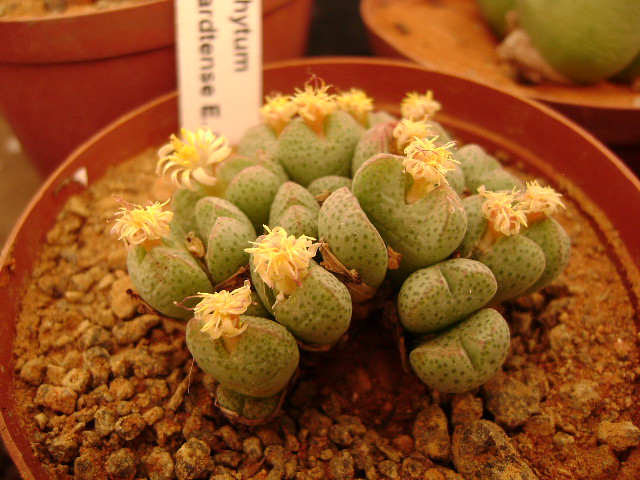The close-up photograph captures a succulent-like plant thriving in a red or rust-colored pot. The pot is positioned at the lower part of the image, extending out of frame, and features rocky, light brown soil. Sprouting from the soil are green, bulbous pods reminiscent of chickpeas or beans, with some showcasing emerging yellow flowers. Not all pods have sprouted yet; roughly half remain unopened. A thin, white label is inserted into the soil, displaying partial text— "Phytum" and "Ardentence" with visible letters above a cut-off section. The background reveals another red pot in the upper left and a larger green plant in a separate pot to the upper right. The setting includes a wooden surface, indicating an arrangement of similar potted plants.